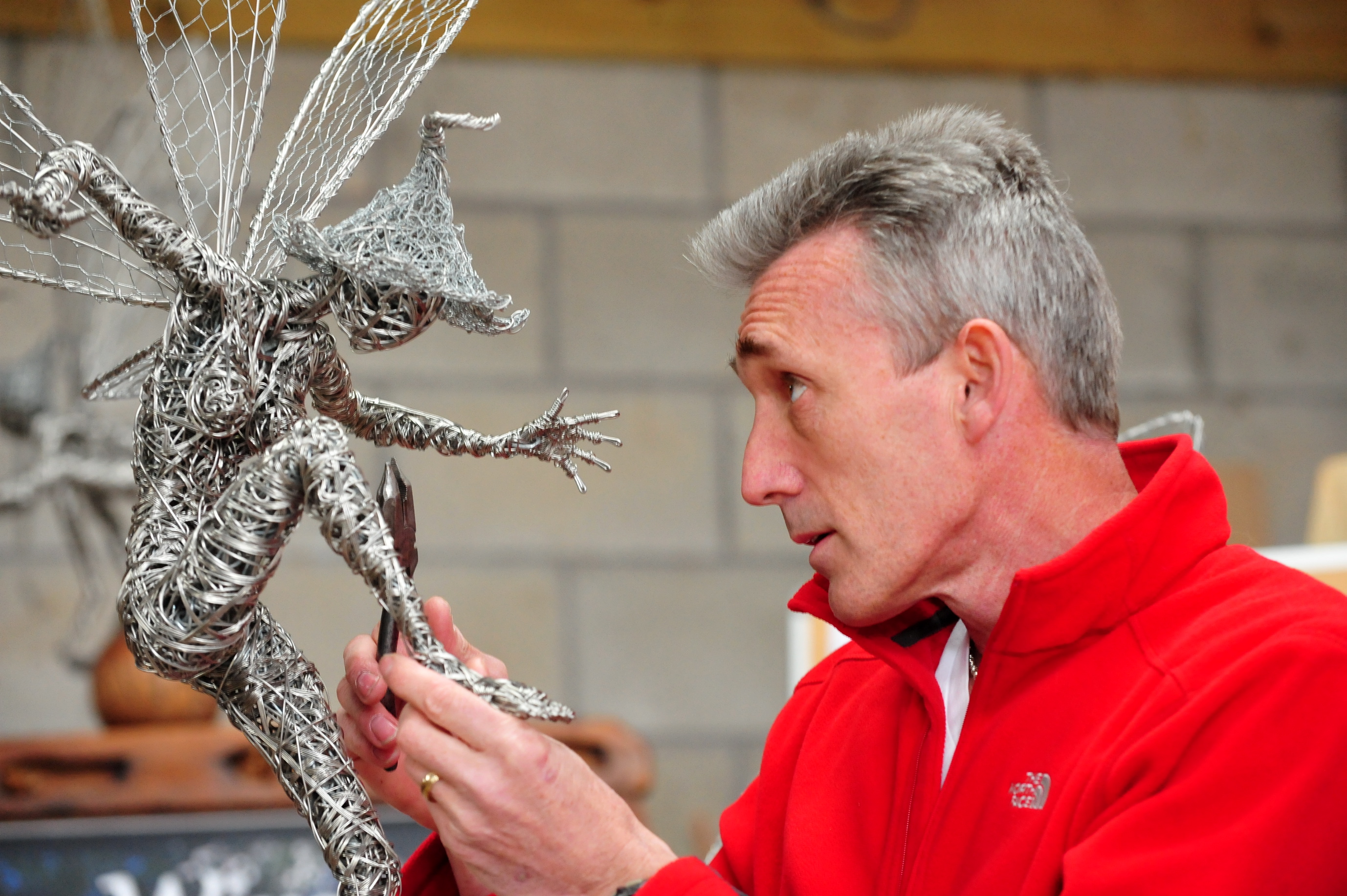A mature white man is carefully crafting a detailed wire sculpture of a fairy-like female figure. He is wearing a red sweater with the collar up over a white shirt, and his gray flat-top hair gives him a distinguished appearance. The man is holding the delicate sculpture, which features intricate details such as a witch hat, raised leg, outstretched arms, and fairy wings, all meticulously formed from thin, wound wire. The scene is set against a cinder block wall with wooden beams above, suggesting a workshop atmosphere. The background includes colors like red, gray, brown, silver, and black, enhancing the industrial feel of the space. The photo captures the man in profile on the right side, intensely focused on the sculpture he holds, with pliers in one of his hands. The overall impression is one of artistic dedication and impressive craftsmanship.